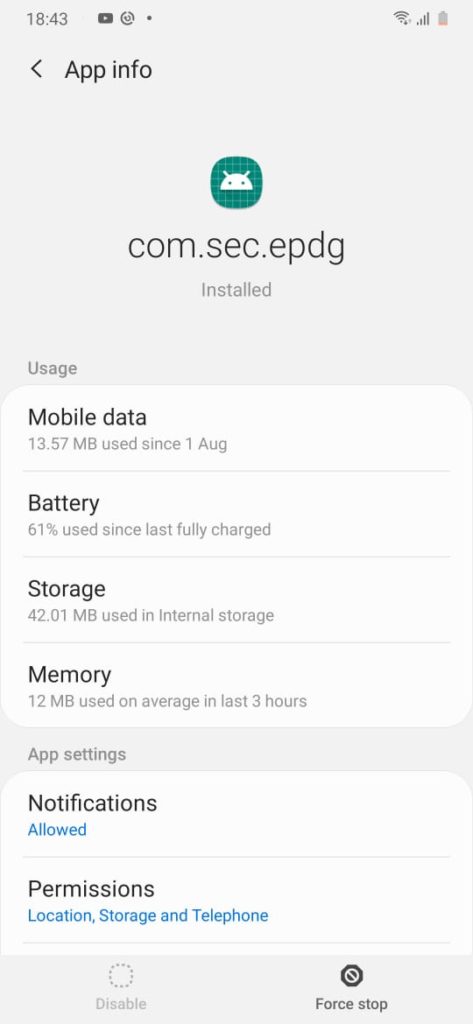This screenshot, taken from a smartphone, features the "App Info" screen at the top, indicated by an arrow pointing left. Below this section, the text "com.sec.epdg" is displayed, denoting the name of the installed application. A green icon portraying a simplified head with two small antennas and two dots for eyes appears above the app name.

Beneath the app name, there is a rectangular section divided into four tabs labeled "Mobile Data," "Battery," "Storage," and "Memory." Diagonally across the screen, a string of capitalized letters, "TERMAR," is prominently printed.

At the bottom of the screenshot, the text "This image is protected" is displayed. Further down, at the bottom section of the app's interface, are two tabs labeled "Disable" on the left and "Force Stop" on the right.